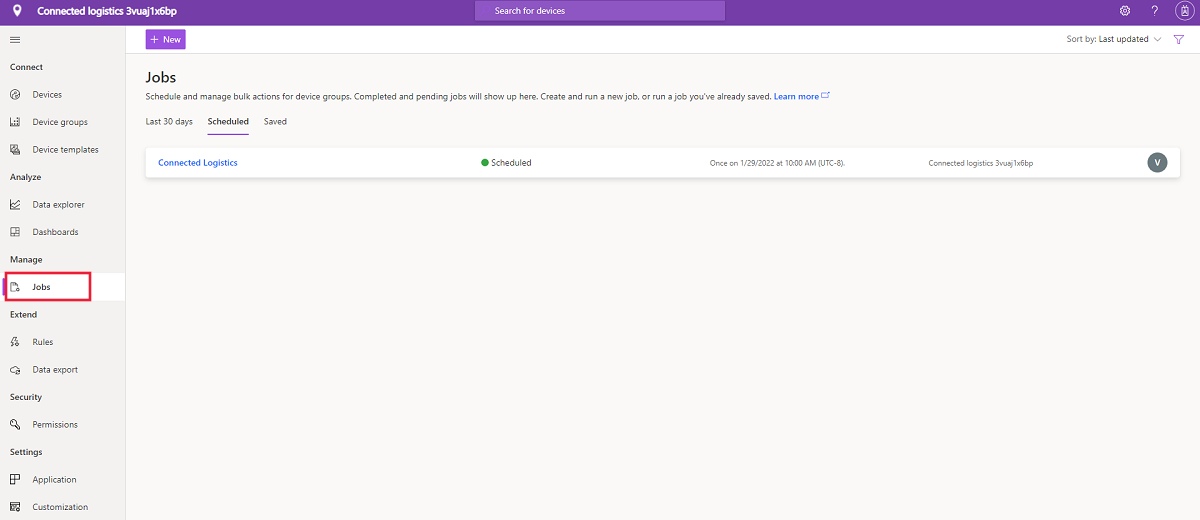This image, sourced from a jobs-related website, prominently features the header "Connected Logistics" in purple text. The design includes a purple toolbar and a purple search bar at the top. The left column presents various options for connectivity, including sections for analysis, management, and security, each meticulously categorized. At the center of the image, the word "Jobs" is displayed, accompanied by a minute and nearly illegible description. A noticeable blue "Learn More" link with a question mark invites users to gather further information. This call-to-action, along with the term "Connected Logistics," is positioned within a white bar, which also contains the subscription option and two other indistinct words. Toward the right end of the white bar, a clickable blue circle hints at additional details upon interaction.